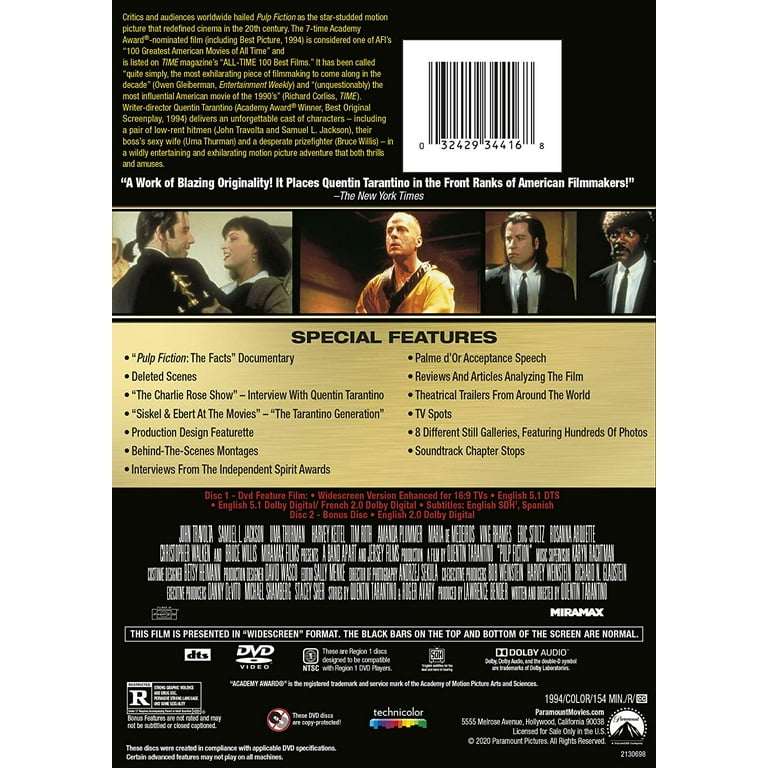This image shows the back cover of a DVD case for the movie "Pulp Fiction." At the top left corner, there is yellow text adjacent to a black and white barcode. Below, a quote from The New York Times in white text reads, "A work of blazing originality. It places Quentin Tarantino in the front ranks of American filmmakers." Beneath this quote, there are three screenshots featuring well-known actors John Travolta, Bruce Willis, and Samuel L. Jackson. The middle section has a light brown background detailing "Special Features" in a black header, followed by a list of these features. Below this section, the background turns black again, featuring small red text and additional white text usually listing the primary creators involved in the film's production. At the bottom, various logos including the DVD symbol, the film's rating, and logos from Paramount Pictures and Technicolor are shown. The cover also notes that the film is presented in a widescreen format, with typical black bars on the top and bottom of the screen.